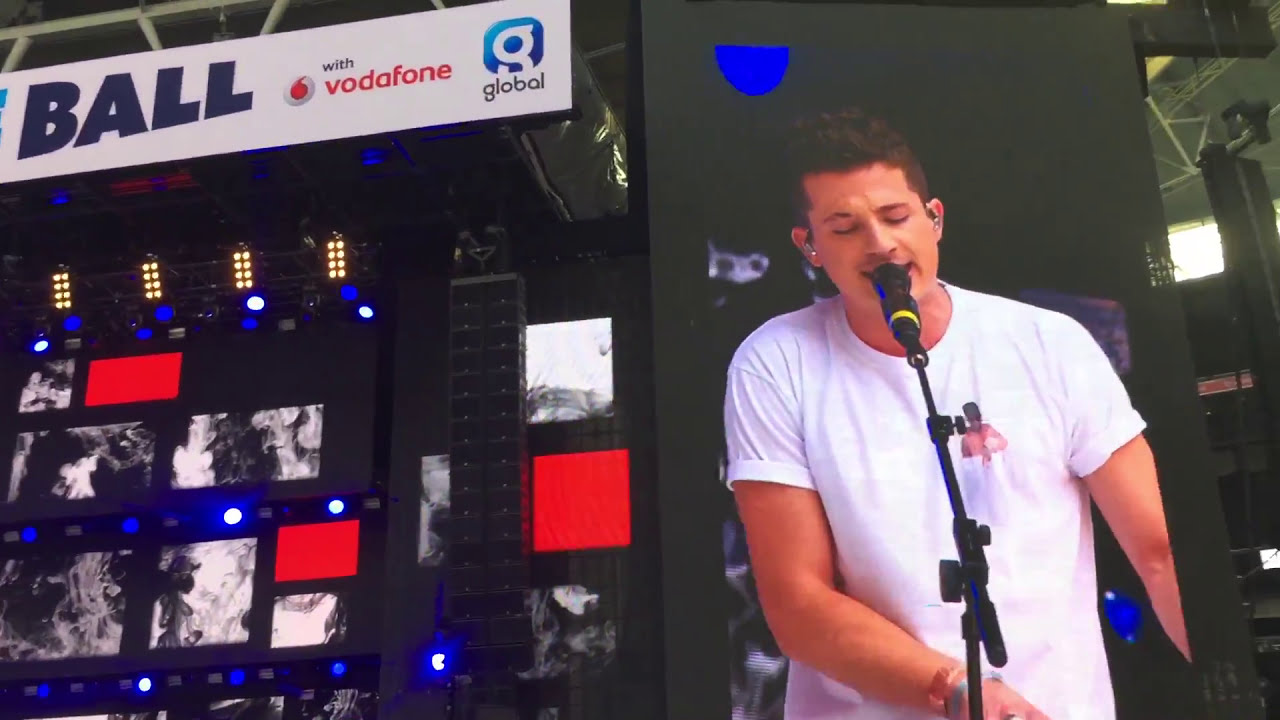The image captures a vibrant outdoor music concert, showcasing a young white male performer, who appears to be singing passionately into a microphone. Positioned slightly to the right of center, the singer, with short dark brown or black hair and wearing a white t-shirt with a distinct red stain near the heart, has his eyes closed and mouth open, fully immersed in his performance. His arms are positioned with the right hand on an unseen object in front of him and the left arm extending to the side.

To the left of the performer, the background features a black wall adorned with color blocks of blue, gray, and red hues. Above this, a sign reads "Ball with Vodafone Global," with "Ball" in navy blue font and "with Vodafone" in lowercase letters. The top left corner hosts lighting fixtures arranged in a pattern, casting blue and white lights that blend with the scene. Multiple monitors and buttons, indicative of the concert’s technical setup, are also present in this area.

The right side of the image includes a screen displaying another person singing on stage, reinforcing the atmosphere of a live musical event. The image is rich with details like various shades of colors – white, black, red, blue, yellow, and gray – contributing to the lively and dynamic setting.